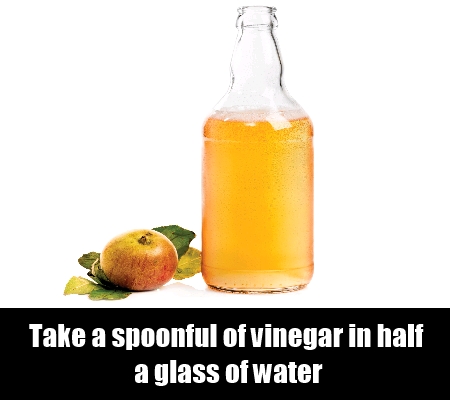The image features a clear glass bottle filled three-fourths full with yellowish orange apple cider vinegar. The bottle has a low cap and holds a mixture of vinegar and water. To the left of the bottle, a red and yellow apple is prominently displayed, surrounded by green leaves. The apple's stem is cut short and points upward. The background is white and segmented into two parts, with a black rectangle at the bottom. Inside the black rectangle, white bold text instructs, "Take a spoonful of vinegar in half a glass of water." This detailed composition highlights the apple cider vinegar bottle and the apple, both framed by leaves, along with the instructional text below.